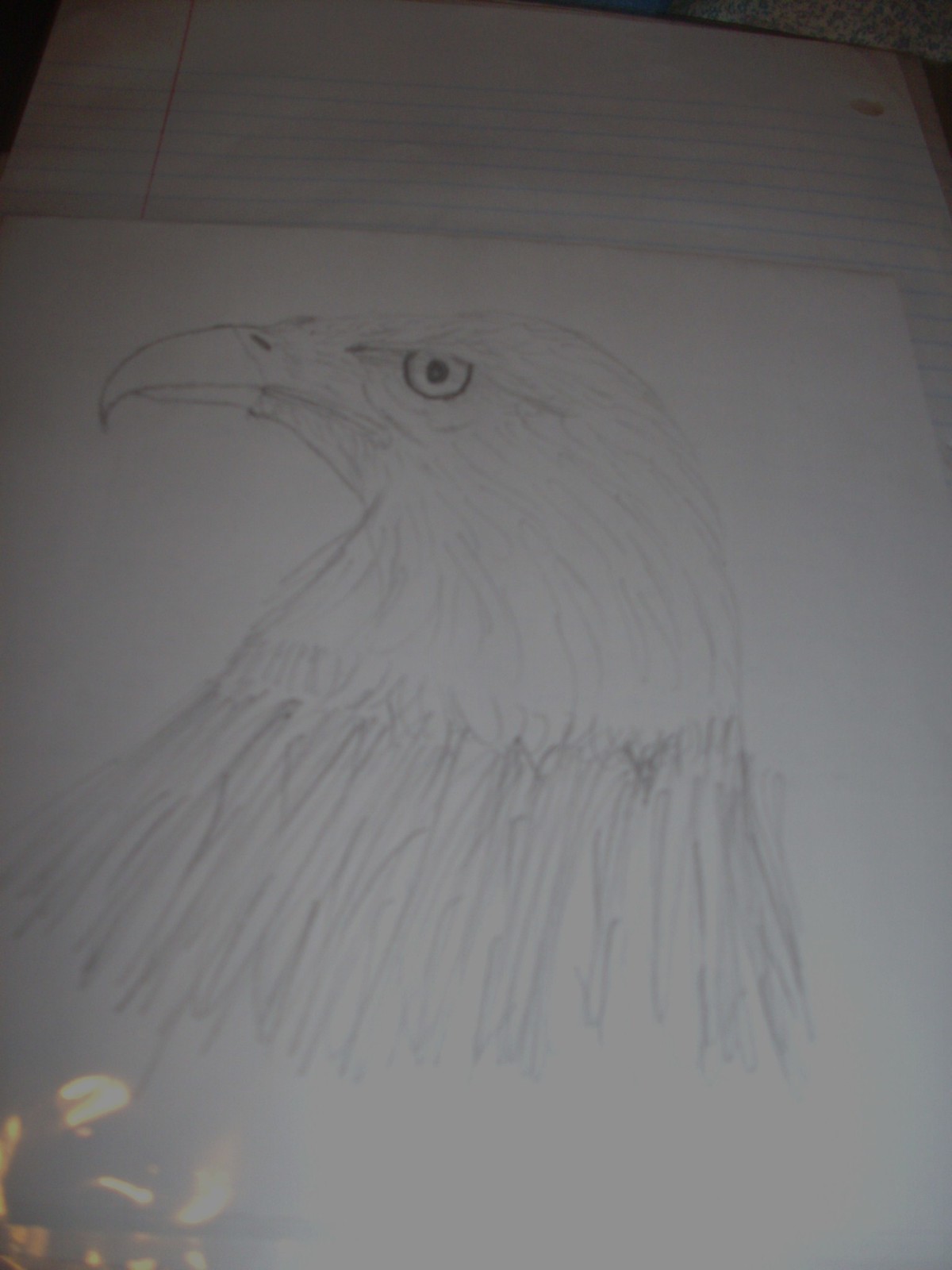This is a meticulously detailed photograph of a hand-drawn pencil sketch, showcasing an American bald eagle. The artwork features the majestic bird in profile, with its gaze directed solemnly to the left side of the page. The artist has skillfully utilized lighter shading to accurately depict the white plumage of the eagle's head, contrasting it sharply against the darker, more intense shading used for the neck feathers. The eagle's eye is rendered with a stern and stoic expression, as if the bird is intently focusing on potential prey, ready to launch into action. The drawing is executed on plain, unlined paper, but it is placed atop a single sheet of standard lined 8.5 by 11-inch paper, providing a subtle, contrasting background that emphasizes the clarity and precision of the eagle sketch. The entire piece is rendered in shades of white and gray, capturing the stark beauty and powerful presence of this iconic bird of prey.